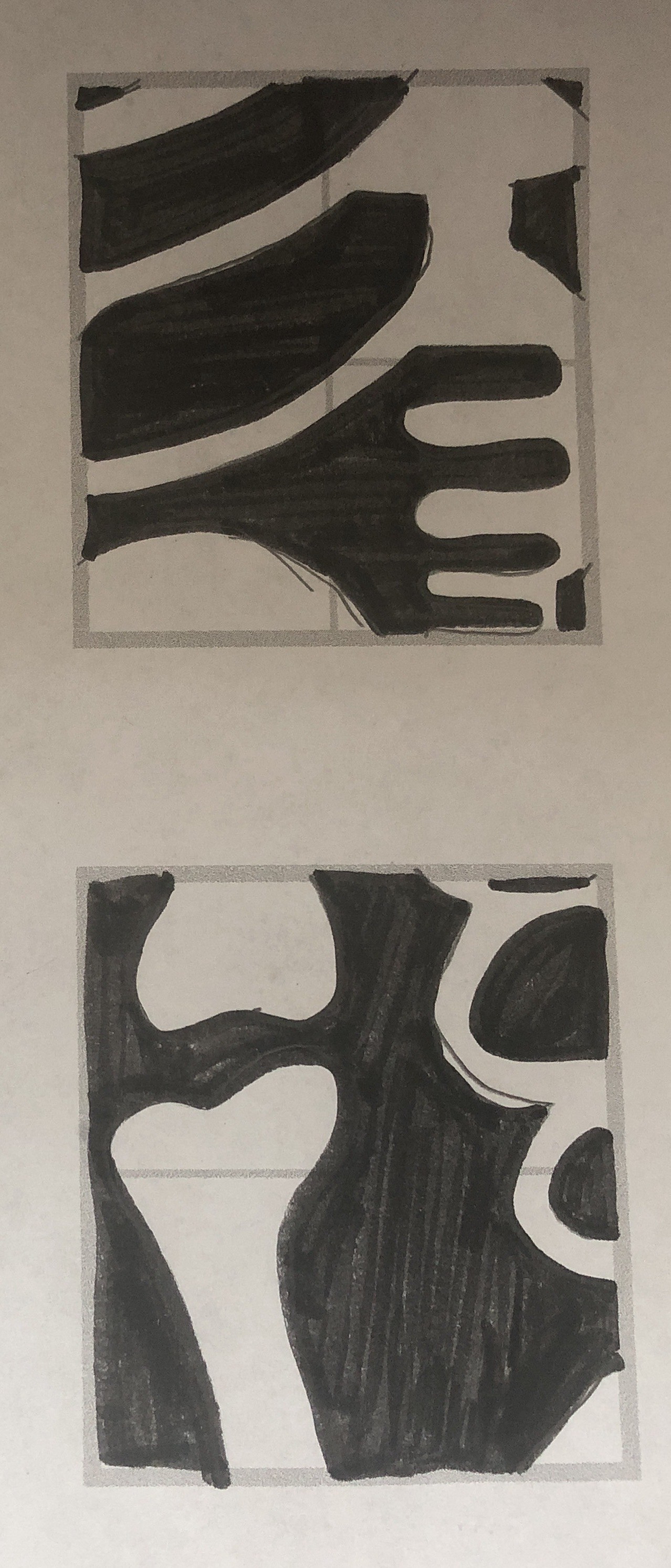This image features two distinct anatomical drawings, both rendered in detail on the same sheet of paper but separated into different sections. The top drawing depicts a complex arrangement of skeletal elements, including a ribcage, shoulder blade, arm, and a fragment of a skull. The artist has meticulously highlighted these components using a black marker, creating bold outlines that emphasize the skeletal structure against a contrasting background. The second drawing, located below the first, showcases a singular elongated bone that arcs gracefully, alongside an abstract shape resembling a figure-eight pattern. This shape, too, is accentuated in black marker, standing out starkly against the white of the paper. The use of negative space ingeniously brings attention to the anatomical details, with the intricate outlines in black creating a striking visual impact. The drawings, while on the same sheet, are clearly distinct, showcasing the artist's skill in both anatomical illustration and creative composition.